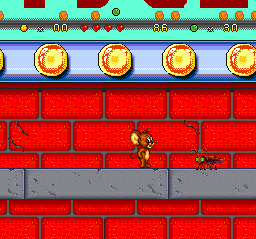The image is a screenshot of a retro Tom and Jerry video game, likely from the 90s. It features Jerry, the little brown mouse, standing upright on a row of gray bricks that stretch horizontally across the screen. Jerry faces an insect-like enemy with antennae and green eyes, which stands at a noticeable gap in front of him. The background is composed of large, cracked red bricks at the bottom two-thirds, transitioning to big, carnival-like round lights against a blue background. Above this are various game interface elements: on the left, a coin symbol followed by "00" in gold; to the right, four red hearts, a green circle with an "X" symbol, and the number "30" in gold. Higher up, the sky is teal-colored, adorned with a row of round orange balls and one distinct green ball. The scene captures the game's nostalgic, pixelated aesthetic, complete with the player statistics and score counters commonly seen in vintage video games.